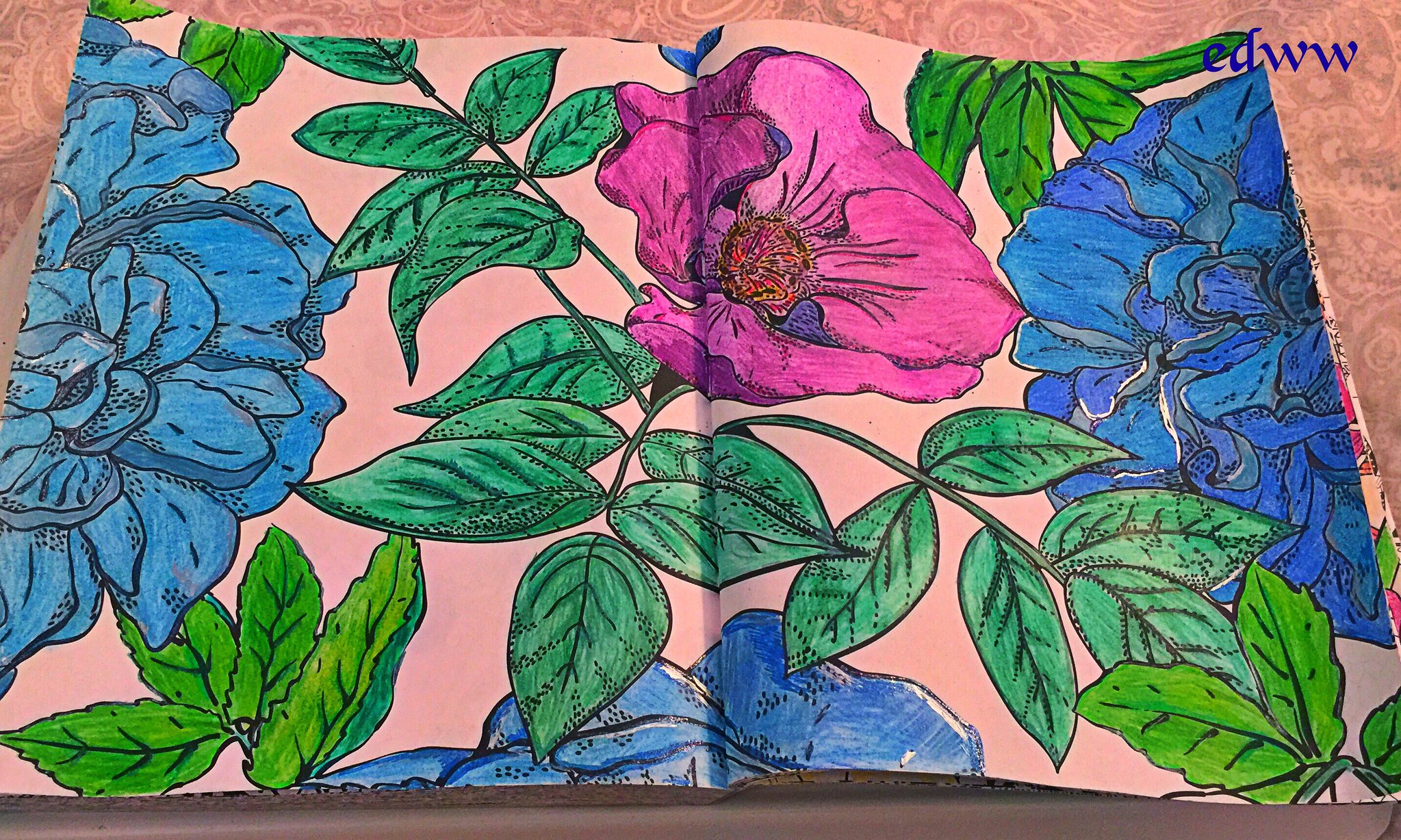This is a detailed color photograph that shows an open coloring book or illustration book laid out on a pink surface, possibly a tablecloth. The pages of the book are opened, revealing a hand-colored illustration that spans both pages. The background of the illustration is a light pink color, adorned with various flowers and leaves. 

At the center of the page sits a prominent purple flower, which is flanked on either side by uniquely styled blue flowers. Additionally, amidst these main flowers, there are several smaller leaves, which are shaded in dark green and teal hues. 

One of the flowers on the right side of the image is partially visible and has petals in shades of dark royal blue and teal. The central flower is notable for its pink petals and a fuzzy yellow center, suggesting pollen. 

The details in the illustration are meticulous, with a harmonious blend of colors—primarily blue, purple, green, and pink—creating an eye-catching composition. There is text visible at the top right of the magazine that reads "EDWW," but no other writing or extraneous elements such as people, animals, buildings, or vehicles are present in the image. The overall dimensions of the image are wider than they are tall.